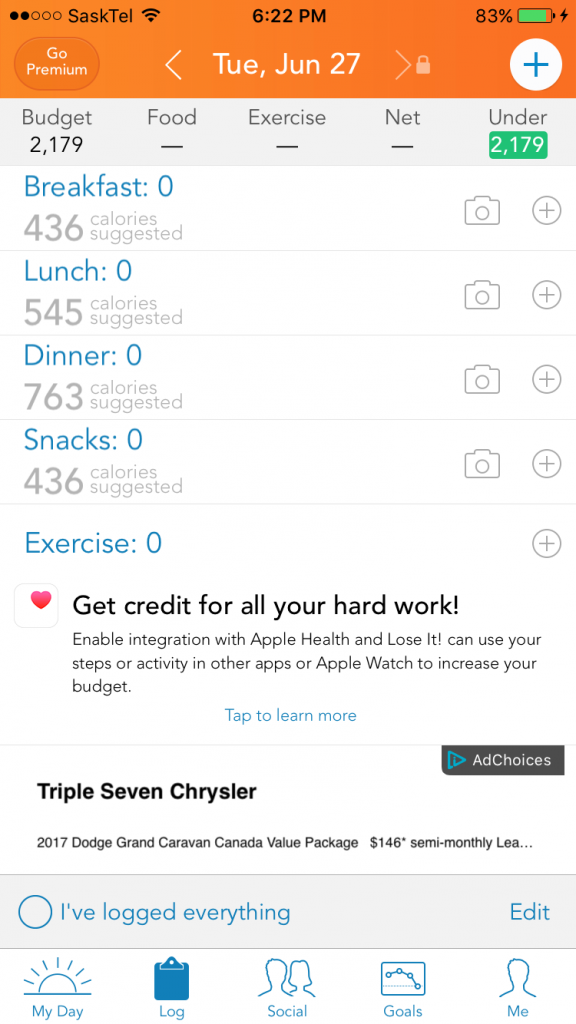The vertical rectangular image displays a smartphone screen showcasing a calorie counter app. At the very top, there's an orange status bar spanning the width of the screen. On the top left, the status bar features four circles, two of which are highlighted to indicate signal strength. Next to the circles, the text "SASKTEL" is displayed in black, followed by a fully lit Wi-Fi indicator. Centrally, the time is shown as 6:22 p.m. In the top right corner, the battery status is indicated by a green battery icon with an 83% charge, alongside a small charging symbol.

Beneath the status bar, there is a white text area featuring the phrase "GO PREMIUM" on the left. Adjacent to this, the date "Tuesday, June 27th" is displayed in white. To the left and right of the date are arrows, with a small lock symbol near the right arrow. On the far right side of this section is a white circle containing a blue plus sign.

The next section consists of an off-white rectangular box with black text. It provides a summary of daily calorie information: "BUDGET 2179", with placeholders for "FOOD," "EXERCISE," and "NET." The phrase "UNDER 2179" is highlighted in a green box. Below this summary, categories for "BREAKFAST," "LUNCH," "DINNER," "SNACKS," and "EXERCISE" are listed in blue text.